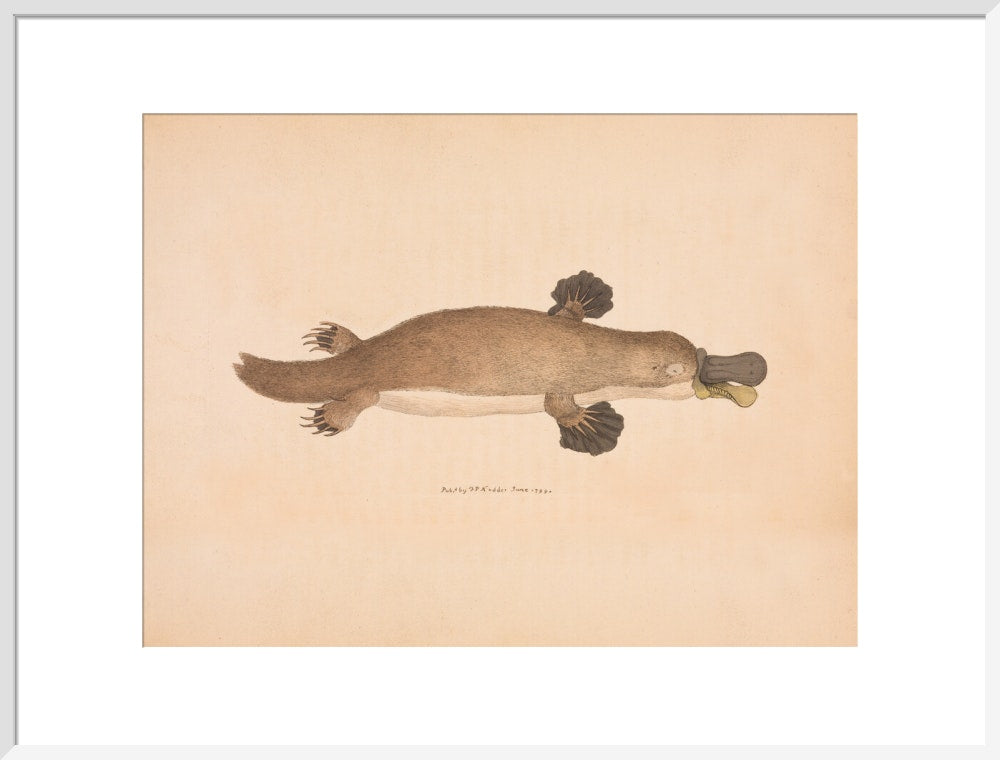This is a framed artwork featuring an old drawing illustration of a platypus, presented on a peach-colored background. The illustration is bordered by white matting and encased in a thin, gray frame. The platypus is depicted in a side view, showcasing its distinctive webbed feet that transition from rodent-like claws in the front to paddle-shaped flippers. Its back legs have sharp, digging claws. The creature's back and legs are brown, while its stomach is a lighter brown or whitish color. The platypus has a long tail and a uniquely colored bill, with a black upper section and a yellow or greenish lower section. The animal appears to be resting on its stomach, facing to the right. The medium of the illustration seems to involve colored pencil, marker, and possibly watercolor, contributing to its detailed, textured appearance. Beneath the platypus, there is some small, blurry, and difficult-to-read text, possibly indicating the month of June.